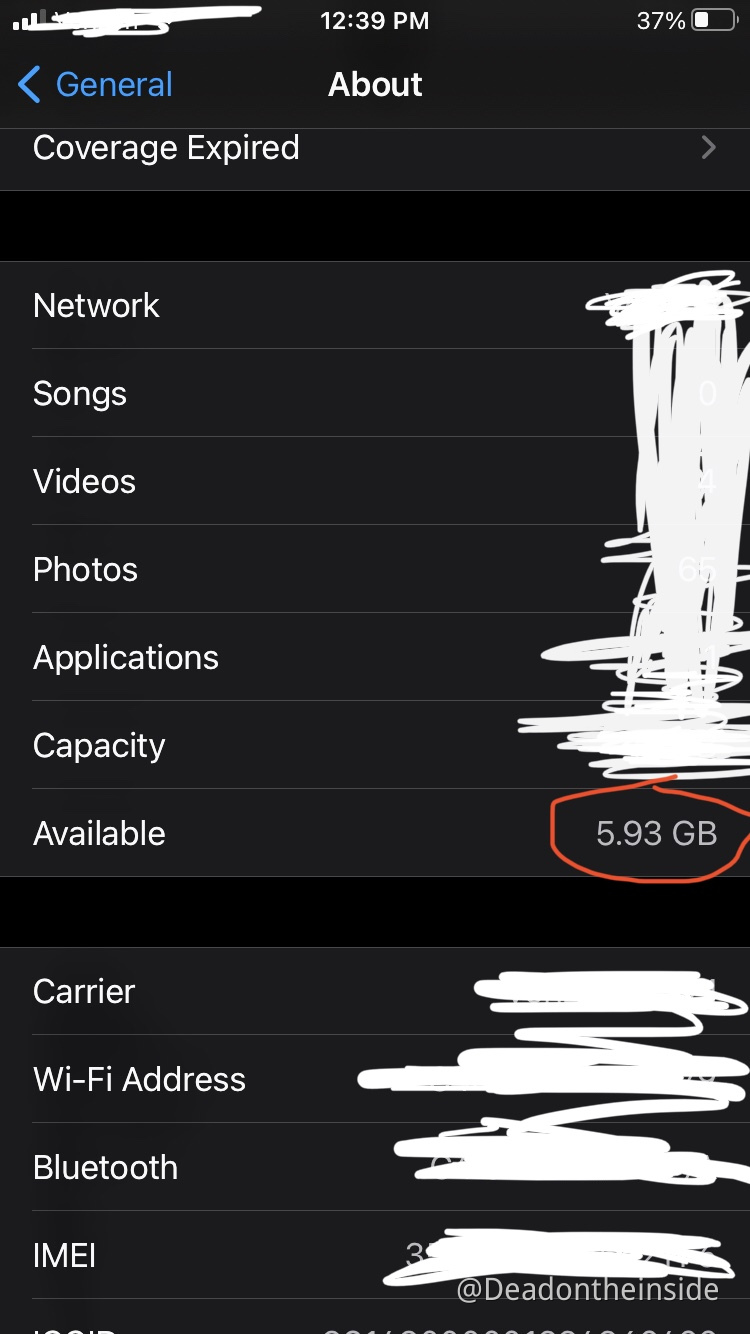The image showcases a screenshot with a predominantly black background in the upper left corner. Notably, certain parts of the image have been intentionally whited out. In the top section, the time "12:39 PM" and battery percentage "37%" are visible. Below this, a blue left arrow icon is displayed next to the word "General" in white text, followed by the option "About" and the phrase "Coverage Expired."

On the left side of the screen, a list of categories is displayed, including "Network," "Songs," "Videos," "Photos," "Applications," "Capacity," and "Available." On the right side, most information is obscured with white scribbles except for the "Available" category, which is circled in red and shows "5.93 GB."

Further down, there are entries for "Carrier," "Wi-Fi Address," "Bluetooth," and "IMEI." Again, much of the text on the right side is obscured by white scribbles, with occasional exceptions revealing partial information. Additionally, some white print at the bottom of the image is cropped off, contributing to the cluttered nature of the visual presentation.